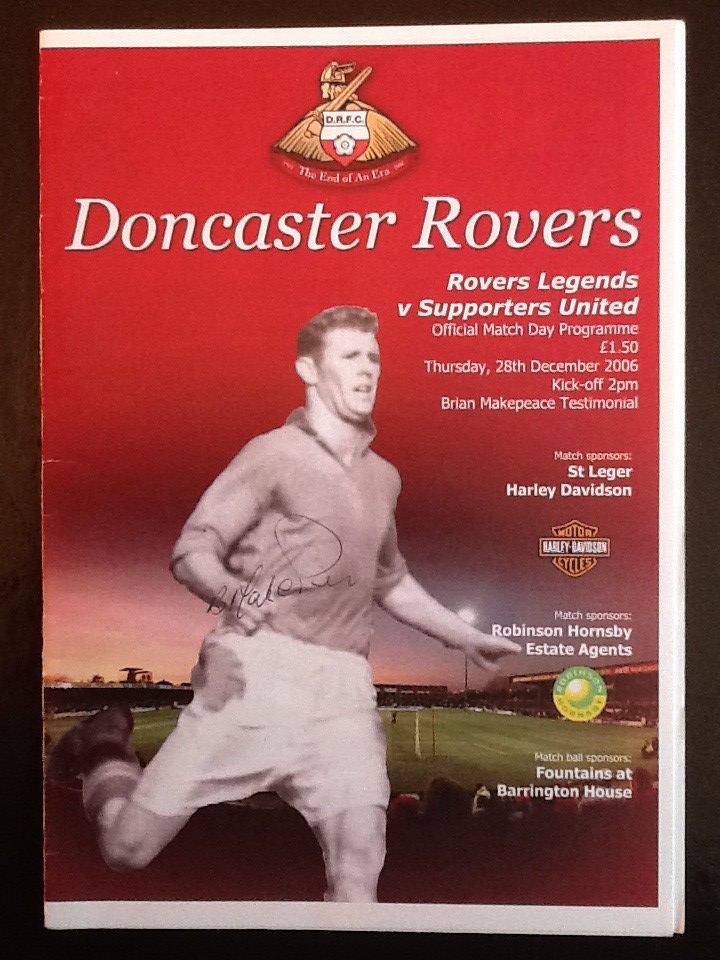This detailed magazine cover in a striking red features a dynamic image of a footballer from the Doncaster Rovers, poised in a running position with his right leg bent back, as if about to kick. He dons a gray top and white shorts, set against the backdrop of a grand stadium. At the top, the cover prominently displays the Doncaster Rovers Football Club insignia—a brown broom-like symbol with accompanying red and white text.

The text across the cover is white, highlighting essential details: the central headline reads "Doncaster Rovers" in bold letters. Below, in the middle of the cover, the footballer's name is written across his chest, though it remains unreadable. To his right, crucial match information is presented: "Rovers Legends versus Supporters United," marking this as the "Official Match Day Program" priced at 1.50 pounds. The event is set for Thursday, 28th December 2006, with a kickoff at 2 p.m., in honor of the "Brian Make Peace Testimonial."

The cover also features various sponsor logos and details:
- Match Sponsors: Robinson-Hornsby Estate Agents, identifiable by their green and yellow logo.
- Match Ball Sponsors: Fountains at Barrington House.
- Additional Sponsors: St. Ledger and Harley-Davidson, marked by the Harley-Davidson Motorcycles logo.

Notably, the cover bears an autograph, characterized by a large, indistinct "B," adding a personal touch to this vibrant and informative magazine cover.